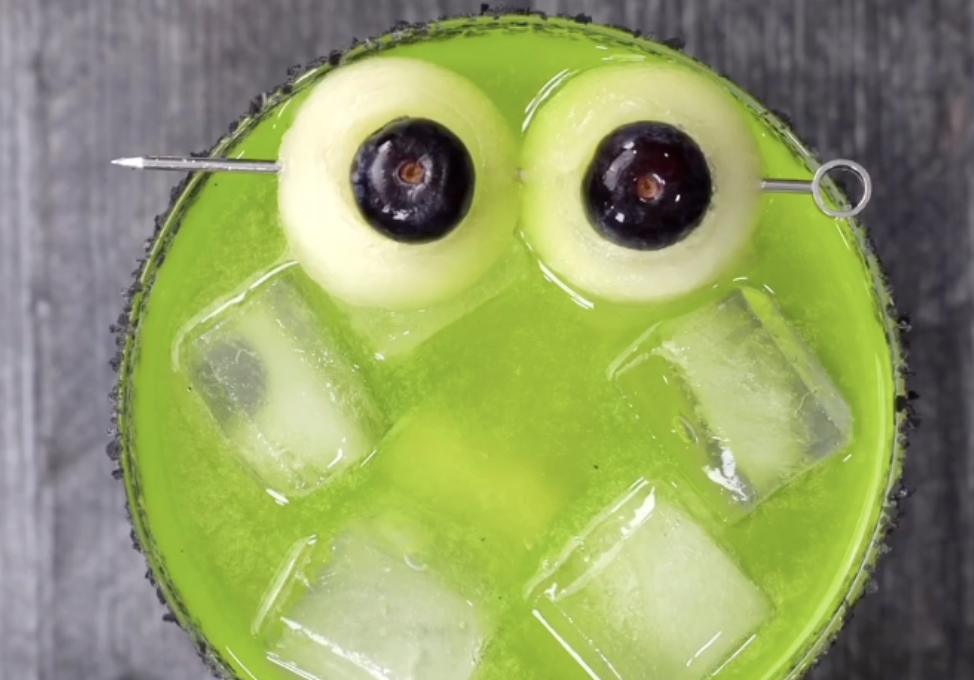This is a detailed photograph featuring a cocktail viewed from the top. The glass is round, containing a neon green liquid that likely resembles a lime-infused soda or a mixed drink. The drink is adorned with four white ice cubes, enhancing its refreshing appearance. Sprinkled along the rim of the glass is a dark material, possibly sugar, salt, or perhaps an herb, implying a seasoned touch to the cocktail.

Resting atop the green liquid is a silver metal skewer piercing through two spherical items that resemble eyeballs. These spheres are melon balls, each stuffed with a single blueberry at their center, giving them an appearance similar to eyes. This creative garnish adds an intriguing visual element to the drink. The cocktail sits elegantly on a gray, wood-grain table, providing a neutral background that emphasizes the vibrant colors of the drink. Overall, this image captures a uniquely adorned and invitingly green cocktail on a minimalist tabletop.